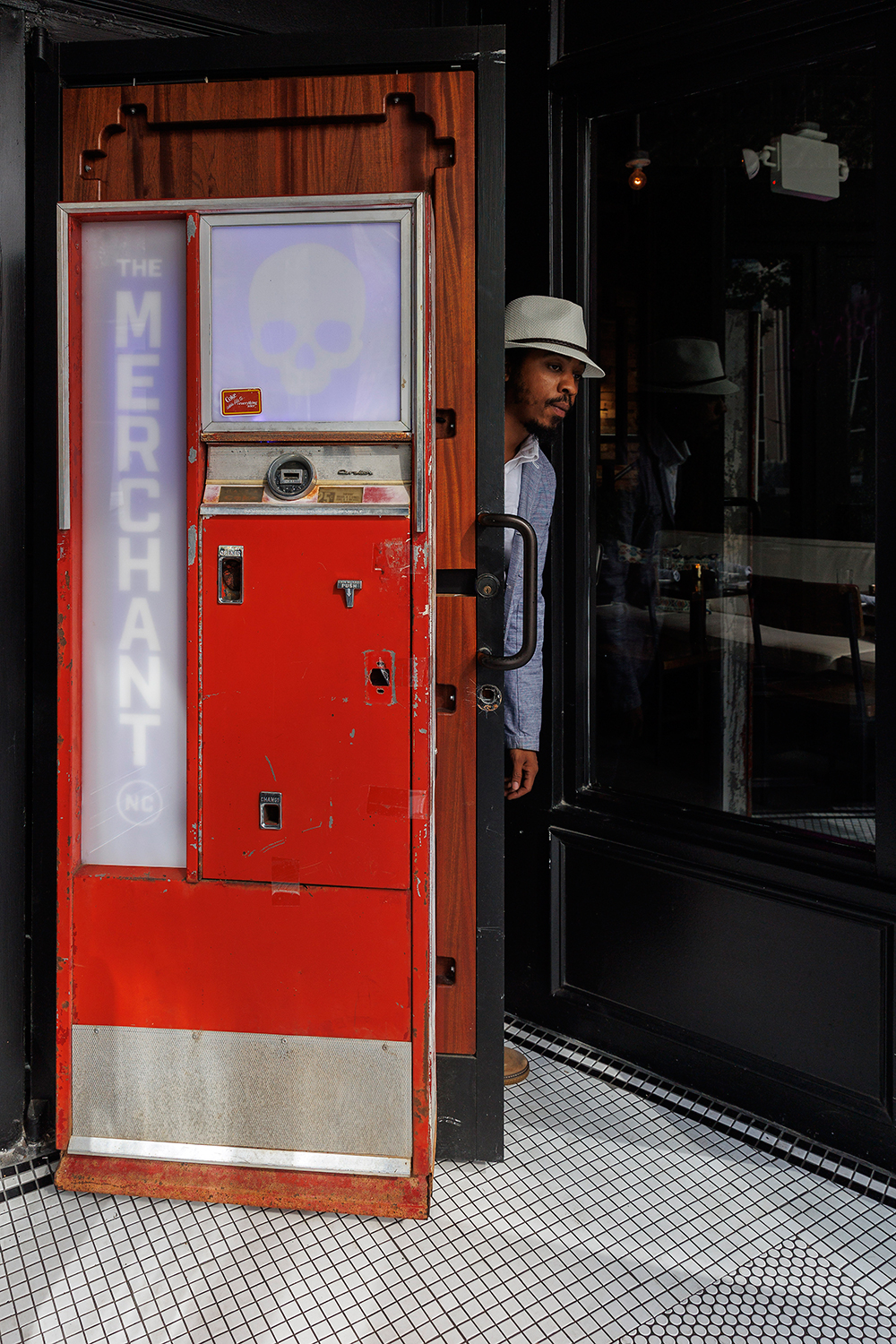The vertically aligned rectangular image depicts the scene inside a store, featuring checkered black and white tiles in small squares covering the floor. A medium brown wooden door, partially open and revealing an African-American man peeking through, takes up a central position. The door is distinguished by a steel plate at the bottom and an old red cover with chipped away paint resembling a worn toolbox, exposing some underlying silver. Above the door's handle is a small square area faintly displaying a skull, while to the left side of the door, a vertical window can be seen with the words "The Merchants" in faded letters.

The man wears a white bucket-style hat with a black ribbon, has dark skin, and short facial hair. His left arm in a blue long sleeve with a white button-down shirt is visible, along with part of his left brown shoe. He peers into the room, which also has a black wall or door on the left side that includes shadows or reflections suggesting the presence of a bench across from it. Behind him, there's another wooden door with black trim, adjacent to the red-covered object labeled "The Merchant," which might resemble an old vending machine with coin slots now unused. The overall setting conveys a sense of deep antiquity and intrigue.